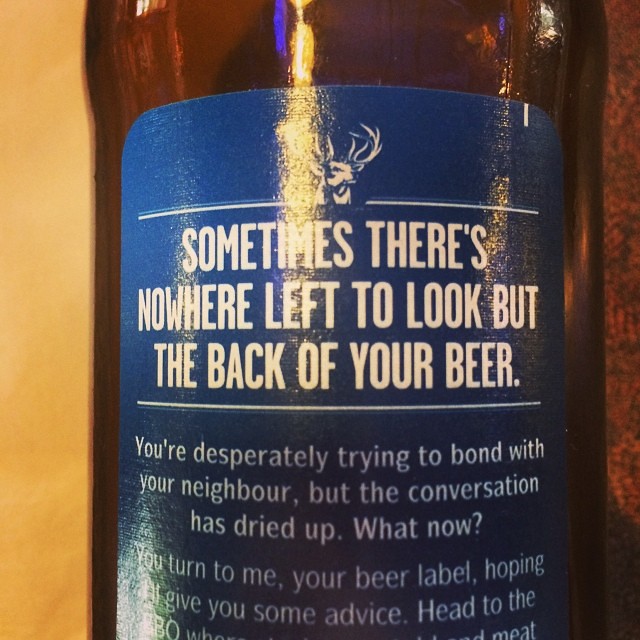The close-up image shows the back of a brown beer bottle with a striking blue label. Dominating the top of the label is an illustration of a deer facing right, with large, imposing antlers outlined in white. Below this, white text reads: "Sometimes there's nowhere left to look but the back of your beer." The text continues with a scenario, "You're desperately trying to bond with your neighbor, but the conversation has dried up. What now? You turn to me, your beer label, hoping to give you some advice. Head to the..." before being cut off. The label appears glossy, with a noticeable sheen reflecting vertically down the center and from the bottom left corner. To either side of the beer bottle is an orange-beige and dark orange-brown background, helping to highlight the bottle itself, which is positioned slightly off-center to the right.